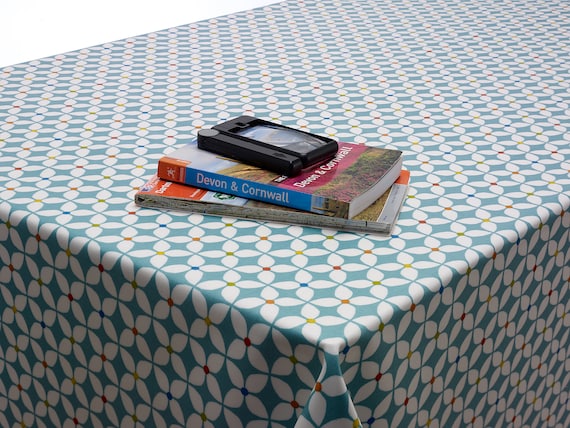The image features a long rectangular table draped in a teal turquoise tablecloth with a geometric pattern. The tablecloth has clusters of four white petals that form flower-like shapes, each surrounding a single colored dot. These dots vary in color, including blue, red, orange, yellow, and green, adding a vibrant touch to the fabric. The tablecloth elegantly drapes over the sides of the table. On the tablecloth, there is a neat stack of books. The uppermost book's title is clearly visible as "Devon and Cornwall," potentially a travel guide to that region in the U.K. Atop this book is a black and gray object, possibly a magnifying glass, which appears to have a screen and may be used to magnify the book below it. Another indistinct book lies beneath the "Devon and Cornwall" book, contributing to the tidy yet intriguing setup on the table.